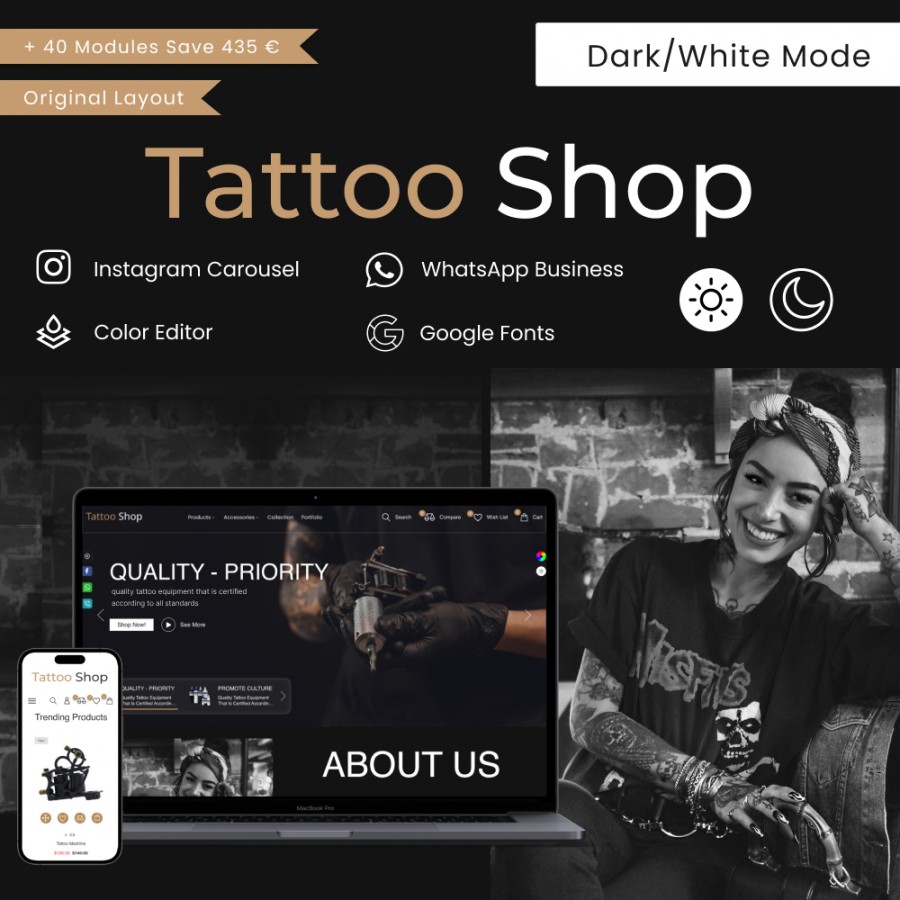This digital advertisement for a product named Tattoo Shop appears to be an intricate flyer designed to showcase a website creation template geared towards tattoo parlors. The image prominently features a woman wearing a black t-shirt with a Misfits band logo, her arms covered in detailed tattoos, and a bandana tied around her head. She stands as a central figure, with a black-and-white aesthetic highlighting her striking body art.

On the left-hand corner of the ad, there's a close-up image of a tattoo artist holding a tattoo machine, displayed on the screen of a MacBook Pro laptop, emphasizing the product's focus on tattoo artistry. An iPhone image at the bottom mirrors the Tattoo Shop interface, offering a glimpse of the user experience on a smartphone. This includes visuals of tattoo-related content and hardware, reinforcing the branding.

The ad touts several features of the Tattoo Shop product with specific text: "Our Quality Priority" and "About Us," presumably underscoring the brand's dedication to high standards. Additionally, it highlights various tools and functionalities such as the Instagram carousel, WhatsApp Business integration, Google Fonts, and a color editor. There is also a mention of a layout feature designed to assist in creating an aesthetic and functional website for tattoo businesses.

Above, a striking gold banner informs potential users of "Plus 40 modules" and a savings claim of "Save $435," suggesting a robust and value-rich offering. A key feature is the "Dark/White mode," providing flexible design options.

In summary, this advertisement for Tattoo Shop compels with its detailed visuals and comprehensive feature set, tailored specifically for tattoo artists and parlors seeking a professional online presence.